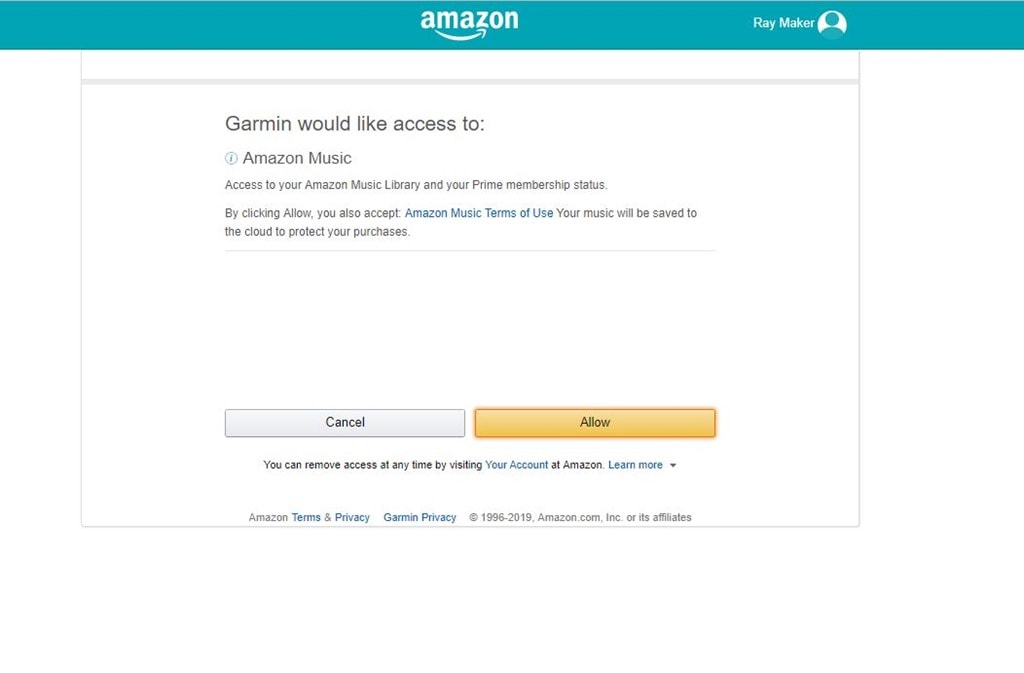The screenshot features a predominantly white background with a horizontal turquoise banner at the top. In the center of the banner, the familiar Amazon name and font are displayed, complemented by the Amazon logo beneath it. To the right of the logo, the user's name, "Ray Maker," is shown, accompanied by a small circular silhouette representing the profile picture.

Below the banner is a large, outlined box with light gray lines. Within this box, the following text is displayed:

"Garmin would like access to:
Amazon Music
Access to your Amazon Music library and your Prime membership status.

By clicking 'Allow,' you also accept Amazon Music's terms of use. Your music will be saved to the cloud to protect your purchases."

At the bottom of the box are two buttons: a gray "Cancel" button on the left and a yellow "Allow" button on the right.